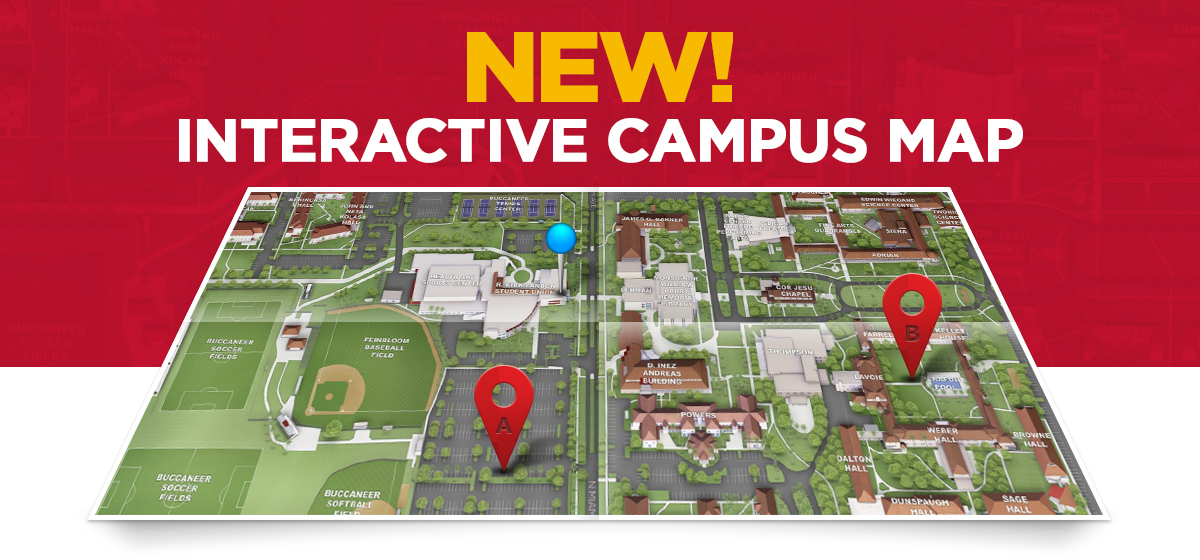The image depicts a detailed and brightly lit interactive campus map prominently displayed on what appears to be an online webpage. At the top of the image, a red banner with subtle lighter shades features the word "NEW!" in large, capitalized yellow letters, followed by "INTERACTIVE CAMPUS MAP" written in smaller, capitalized white letters. The map itself is predominantly green with various markers: red pins labeled A and B, and a blue pin indicating the viewer's current location in the Student Union area. The pin marked A points to a parking lot, while B highlights the pool. Surrounding these key points are various campus landmarks including a baseball field, soccer fields, a softball field, and several buildings such as the D and S Andre Building, Powers Hall, the Barrier Building, Corgesu Chapel, and Weber Hall. The map clearly details roads, athletic fields, dormitories, and other notable locations, providing a comprehensive guide to navigating the campus.